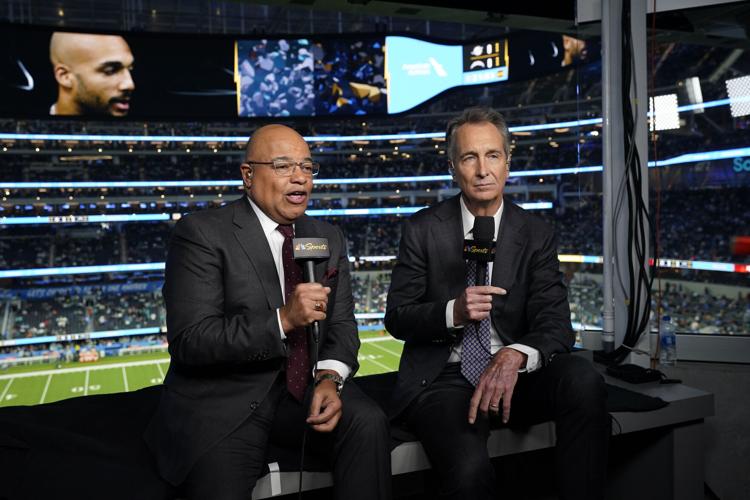This image captures a live sports event broadcast taking place in an announcer box at a stadium, likely in the U.S. The photograph shows two middle-aged sports commentators in mid-action, facing away from the photographer and towards an off-screen camera. The commentator on the left is an African-American man wearing a stylish charcoal suit with a white shirt and a burgundy tie with white dots. He accessorizes with a silver wristwatch, glasses, and an earpiece in his right ear. Holding a microphone featuring the NBC peacock logo and the word "sports," he appears to be speaking. 

The commentator on the right is a Caucasian man dressed similarly in a dark suit, white shirt, and a striking blue checkered tie. He too holds a matching NBC sports microphone. The setting behind them reveals a crowded stadium with blurry outlines of numerous spectators and a field that could be either an American football or soccer pitch, indicated by the visible 50-yard line.

Above them loom large screens or jumbotrons, one displaying the enlarged image of a bald man with a mustache and beard, recognizable by a Nike swoosh, likely a player. The backdrop includes an array of cabling, hinting at the technical setup required for televised broadcasts, and a bottle of water on the right, emphasizing the live, ongoing nature of their coverage. The overall color palette is subdued, dominated by greys and dark tones, lending a professional and focused atmosphere.